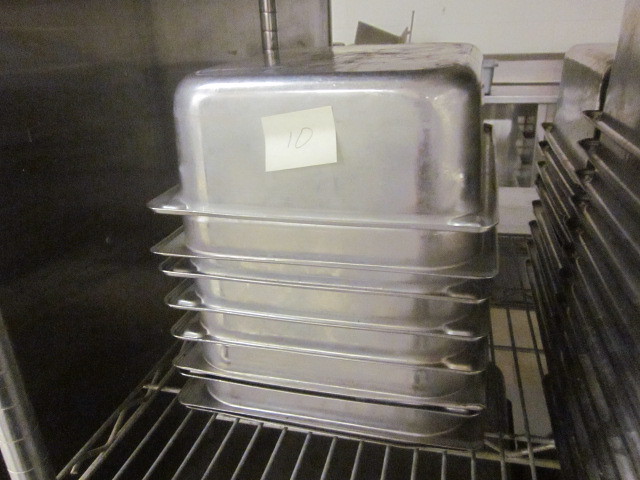A detailed indoor photograph showcases a setting with a sleek, silver metal backdrop on the left-hand side. In the foreground, there is a thick silver metal grate upon which ten large, rectangular stainless steel food holding bins are neatly stacked upside down. The bins vary slightly in size, and each is made of shiny stainless steel, likely intended for use in a steam table to keep food warm. The topmost bin features a white sticky note with the number '10' written in pencil. On the right-hand side of the image, a white wall with a window is partially visible, and the stack is placed inside a stainless steel cart designed to hold multiple shelves, evident from the visible shelf holders on the sides.